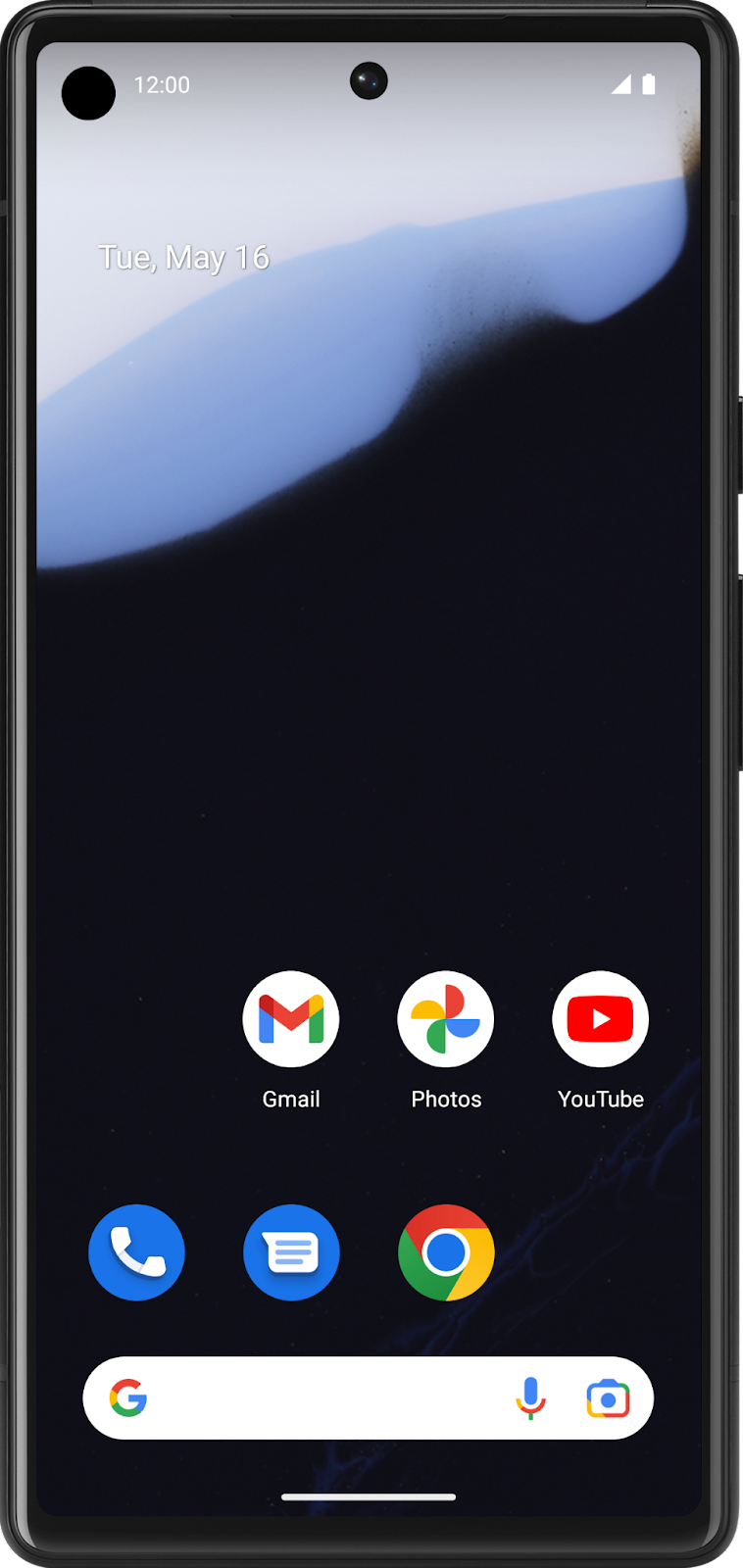This image features a black cell phone centered against a plain, white backdrop. The phone's screen is predominantly black, with a transparent section in the upper left corner displaying the time as "12:00". Adjacent to the time, the text reads "TUE, May 16th". In the upper right corner, signal and battery icons are visible.

Towards the bottom of the screen, the Google search widget is prominent, accompanied by an Android swipe-up line. The home screen is organized into a grid with six app icons. The top row contains the Gmail app, identified by a multicolored "M", the Google Photos app, and the YouTube app. The second row has four available slots, but only three are occupied: a phone app icon, a blue-text message app icon, and the Google browser icon.

The layout and colors of the icons and structure of the screen provide a detailed snapshot of a typical smartphone home screen.